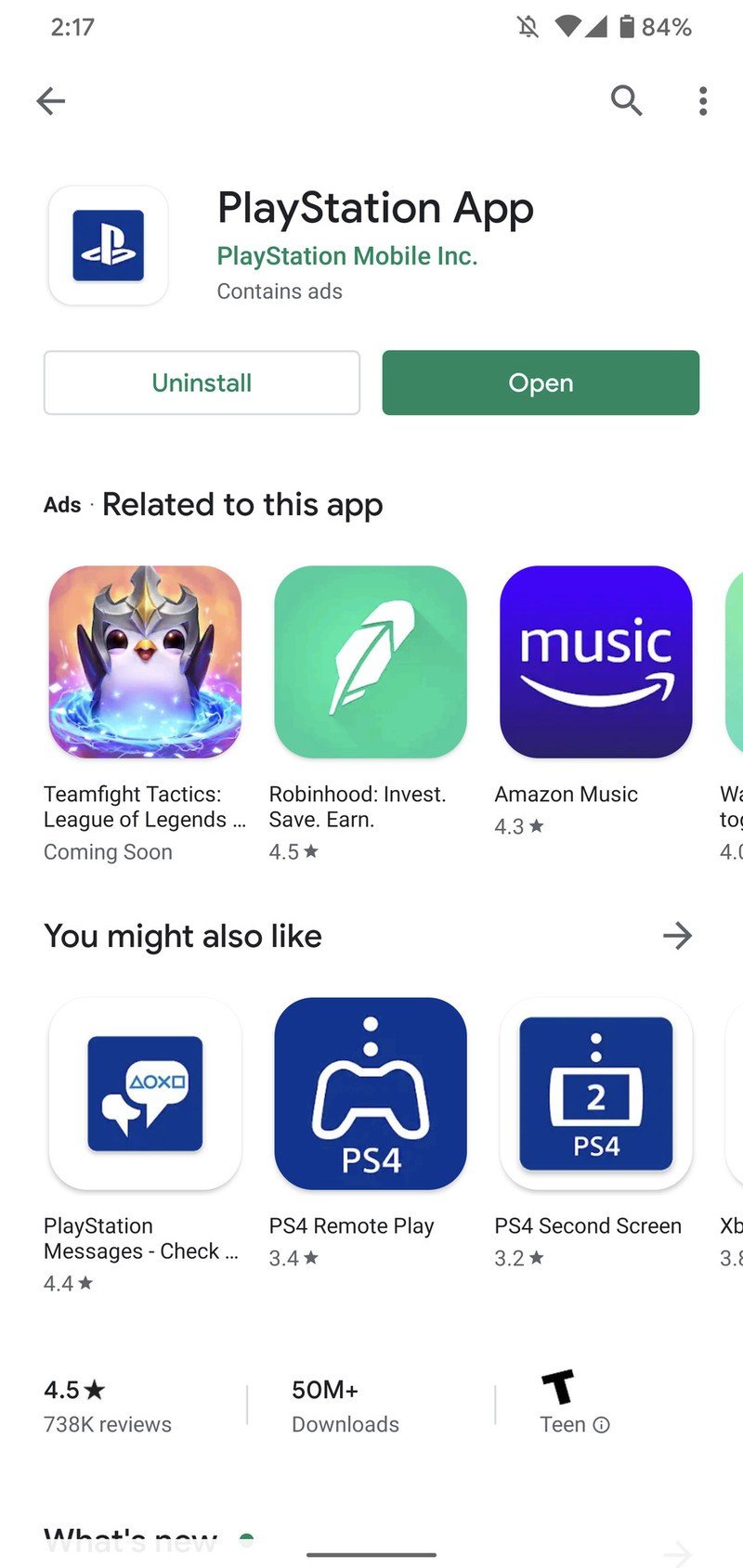This image captures a screenshot from a mobile device displaying a web page for the PlayStation app. The PlayStation logo, characterized by a stylized letter "P" on a blue square background, is prominently placed in the upper left corner. To the right of the logo, the words "PlayStation app" are displayed. Directly below this text, on the left side, is the "Uninstall" button, distinguished by its green text. Adjacent to this, on the right side, is the "Open" button, set against a green background and equally highlighted in green. 

Beneath these buttons, the phrase "Ads related to this app" indicates the section devoted to advertising. Below this, a grid of six app icons is presented, organized into two rows with three icons each. Beginning with the top-left icon, there is an image of a small bird adorned with a gray crown on its head.